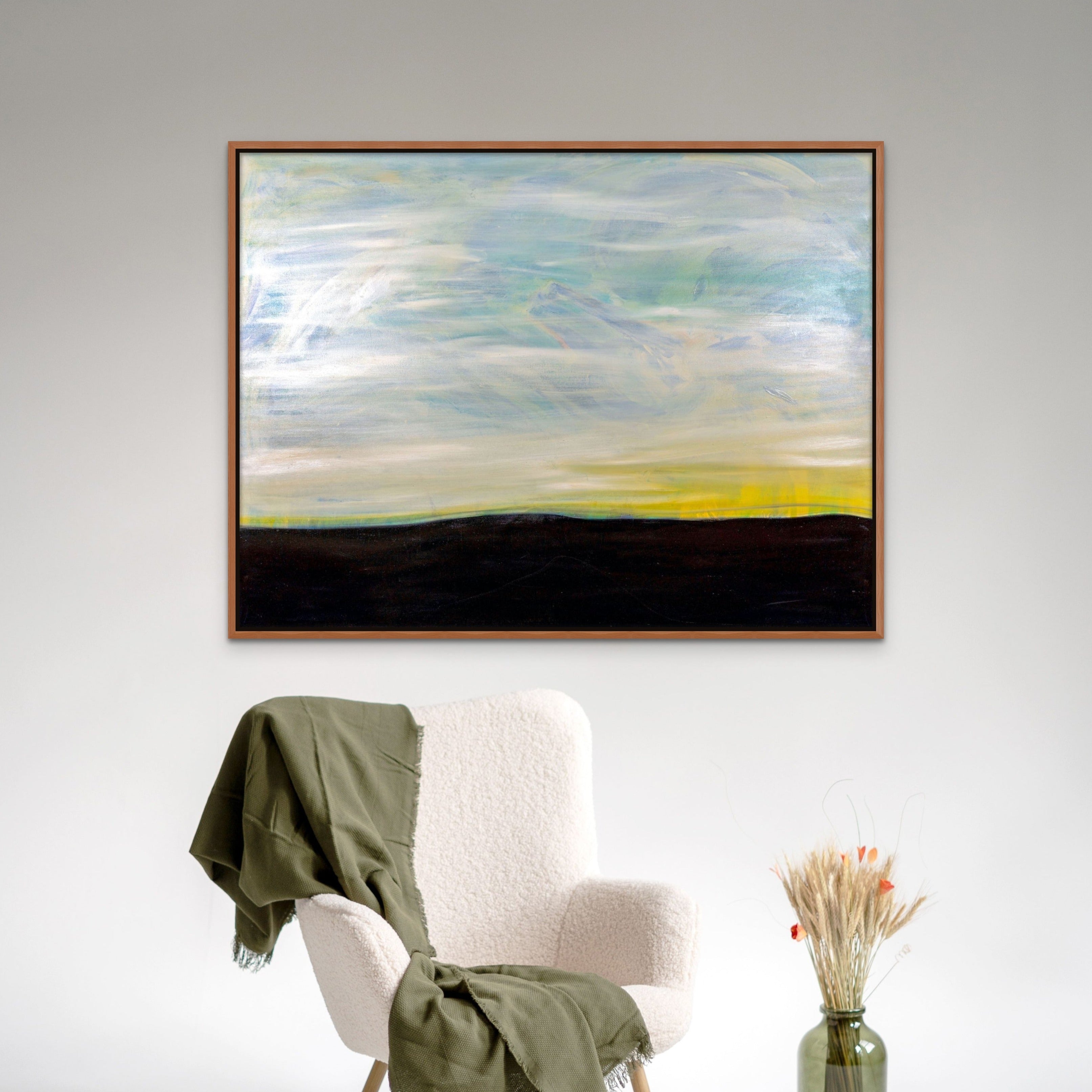The photograph captures a minimalist and well-designed section of a room. Prominently featured is a fluffy white chair with angled wooden legs, draped gracefully with a high-quality army green throw. Adjacent to the chair, a sleek glass vase holds a striking arrangement of dried white pampas grass, adding a natural element to the scene. Dominating the background is an abstract painting encased in a dark pine-colored frame with a subtle black outline. The artwork, which occupies about a third of the photograph, depicts swirling blue and white hues blending into yellow and black, evoking a stylized landscape sans realism. The setting, characterized by its neat and intentionally arranged aesthetic, suggests a carefully staged scene likely meant for showcasing home decor. The backdrop is a white wall, which slightly darkens from the bottom upward, enhancing the overall visual contrast and composition of the room.